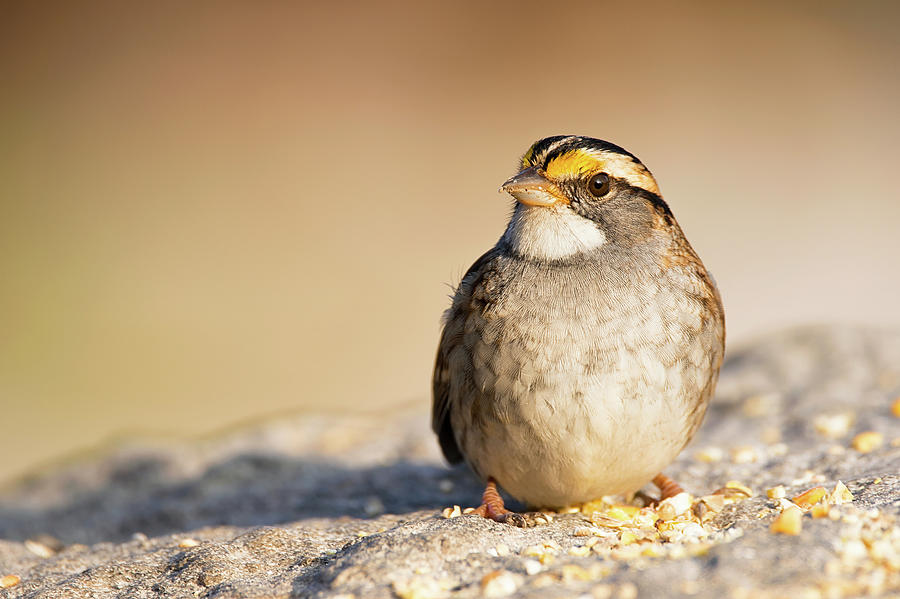This photorealistic image captures a detailed close-up of a small, fluffy chickadee perched on rocky ground. The bird, with its light gray beak and pale orange feet, stands alert near a scattered pile of birdseed situated in the lower right corner of the foreground. Its round body is adorned with brown eyes and a soft yellow patch just above the beak. White feathers are visible under its chin, blending seamlessly into its gray chest. The background, a blurred beige hue, adds an intriguing depth to the scene, suggesting a sandy beach setting while maintaining focus on the intricately detailed bird in the foreground.